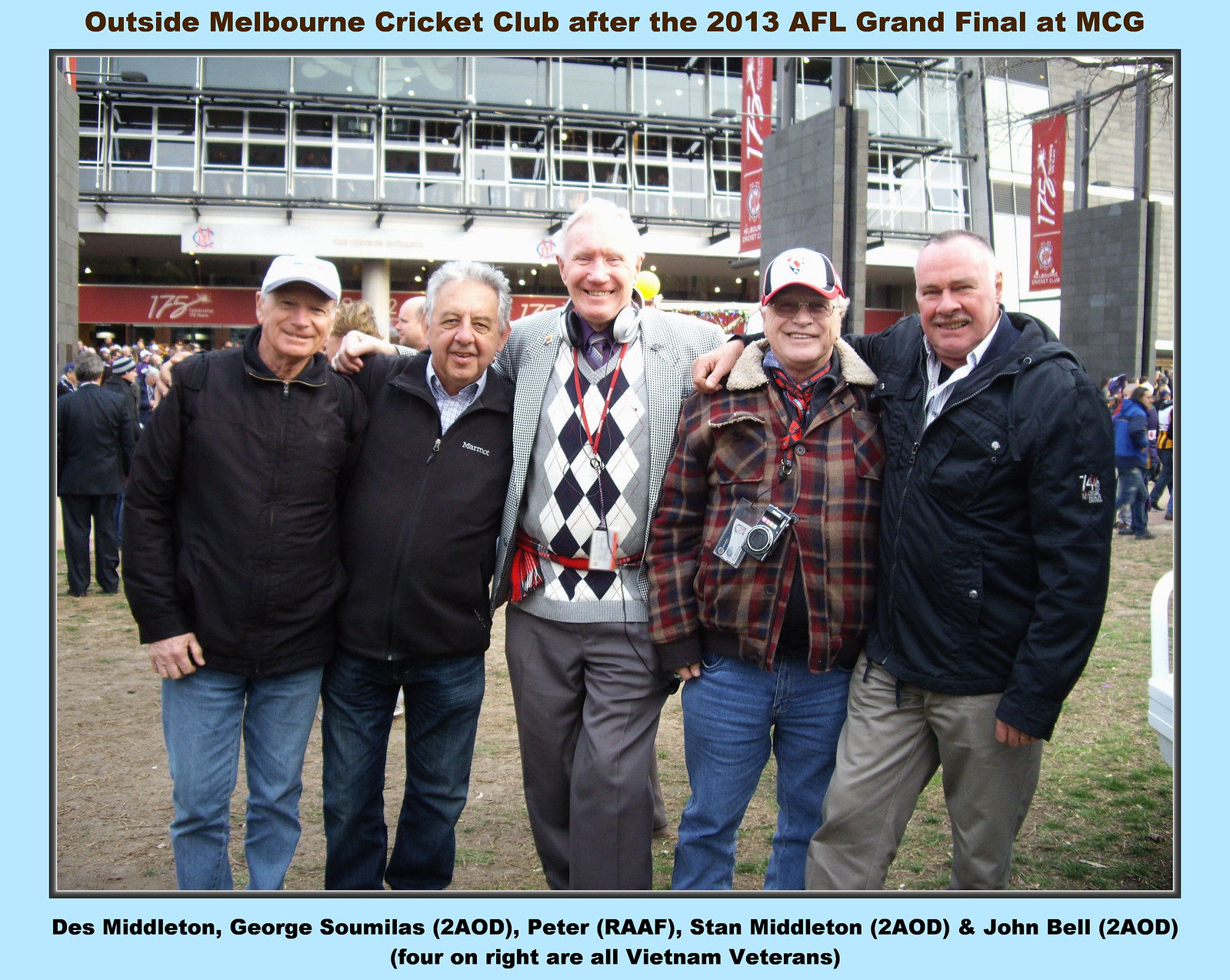This photograph captures a lively moment featuring five middle-aged to older gentlemen posing together affectionately, with their arms wrapped around each other’s shoulders. They are standing shoulder to shoulder, close together, dressed in casual but neat attire appropriate for their age. The gentleman on the far left is wearing a white cap, a black jacket, and blue jeans. Next to him, the second man is also dressed in a black jacket and blue jeans, with white hair and a clean-shaven face. The tallest man standing at the center sports a gray blazer over a patterned V-neck sweater and a shirt, with headphones around his neck and gray pants. Beside him is another man in a checkered jacket, donning a cap, a camera hanging from his neck, and an ID card, paired with blue jeans. The last man on the right has minimal hair, a black jacket over a white shirt, and light gray trousers.

They are set against the backdrop of an outdoor area in front of a stadium, likely the Melbourne Cricket Club, given the visible glass windows and bustling crowd in the background. The men appear to be enjoying the cool weather, as indicated by their heavier jackets. Above the photograph, within a blue border, a heading reads: "Outside Melbourne Cricket Club after the 2013 AFL Grand Final at MCG." Below the photograph, also in a blue border, the names of these gentlemen are listed: Des Middleton, George Sumilas (2AOD), Peter Raaf, Stan Middleton (2AOD), John Bell (2AOD). It further notes that the four men on the right are Vietnam veterans. The camaraderie and shared history among these men are evident in their smiles and congenial posture.